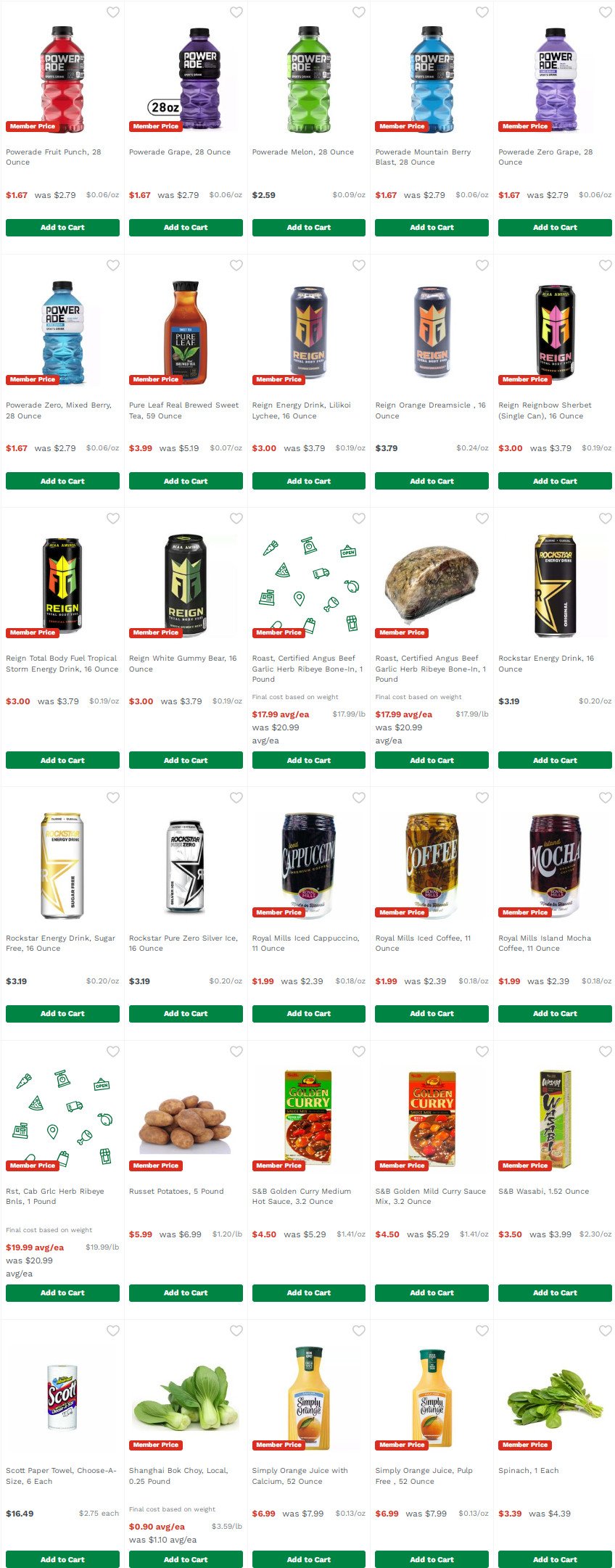A detailed supermarket search results page is displayed in a 5 by 6 grid layout showing various products. At the top row, multiple listings of Powerade are visible in an array of colors including red, purple, green, and blue. Adjacent to some listings, a small red marker labeled "member price" is present, albeit difficult to read due to its size. Below each product, prices are indicated either in red or black text. 

A green "Add to Cart" button is located beneath each product entry. Apart from Powerade, the search results showcase a variety of items including Rain power drinks, a loaf of bread, Rockstar energy drinks, and an assortment of cappuccino and coffee beverages. One entry includes products with unclear icons. Other items found in the grid are nuggets or potatoes, products labeled as curry, orange juice, and a selection of vegetables, including bok choy.